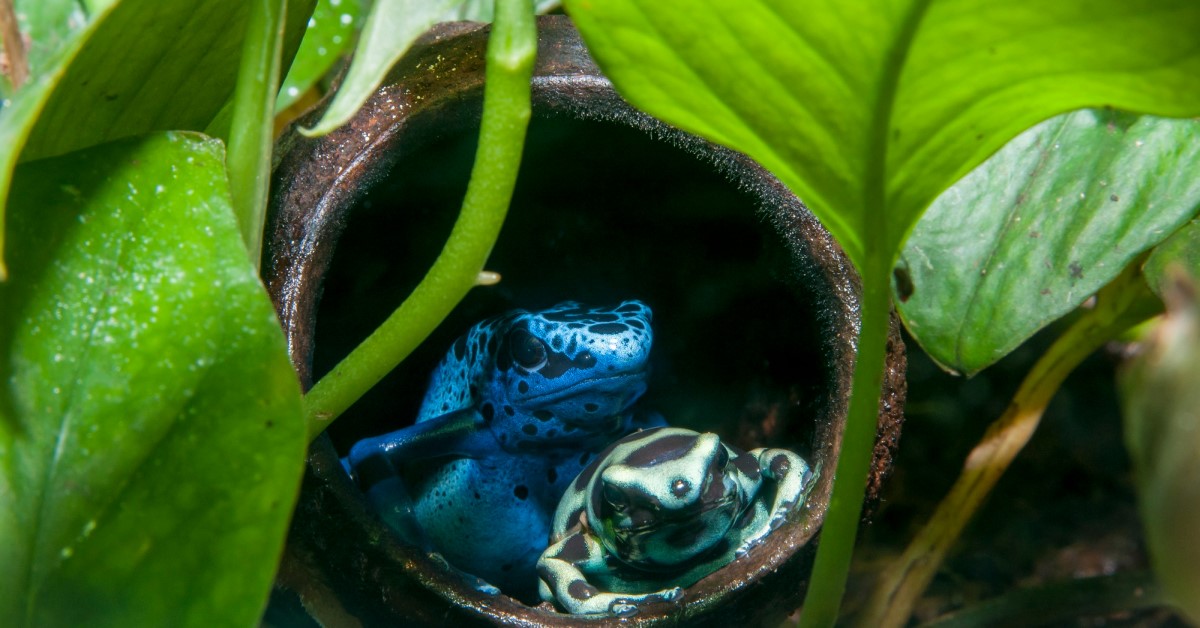The image depicts a natural outdoor scene, likely in a rainforest, illuminated by daylight with a slight brightness. Dominating the picture are vibrant green leaves with some exhibiting brownish or yellowish hues, indicative of moisture due to visible droplets. The leaves frame a circular, pipe-like hollow, black on the inside with a brown exterior. Inside this hollow are two frogs; the one on the left is brightly colored in blue with black spots, while the frog to the right and slightly beneath it is a vivid seafoam green, also adorned with black spots. The frogs appear to be seeking shelter within this circular hollow. The scene captures a rich, verdant environment with detailed, folding leaf faces and thin, green stems, creating an immersive glimpse into a lush, possibly rainforest habitat.